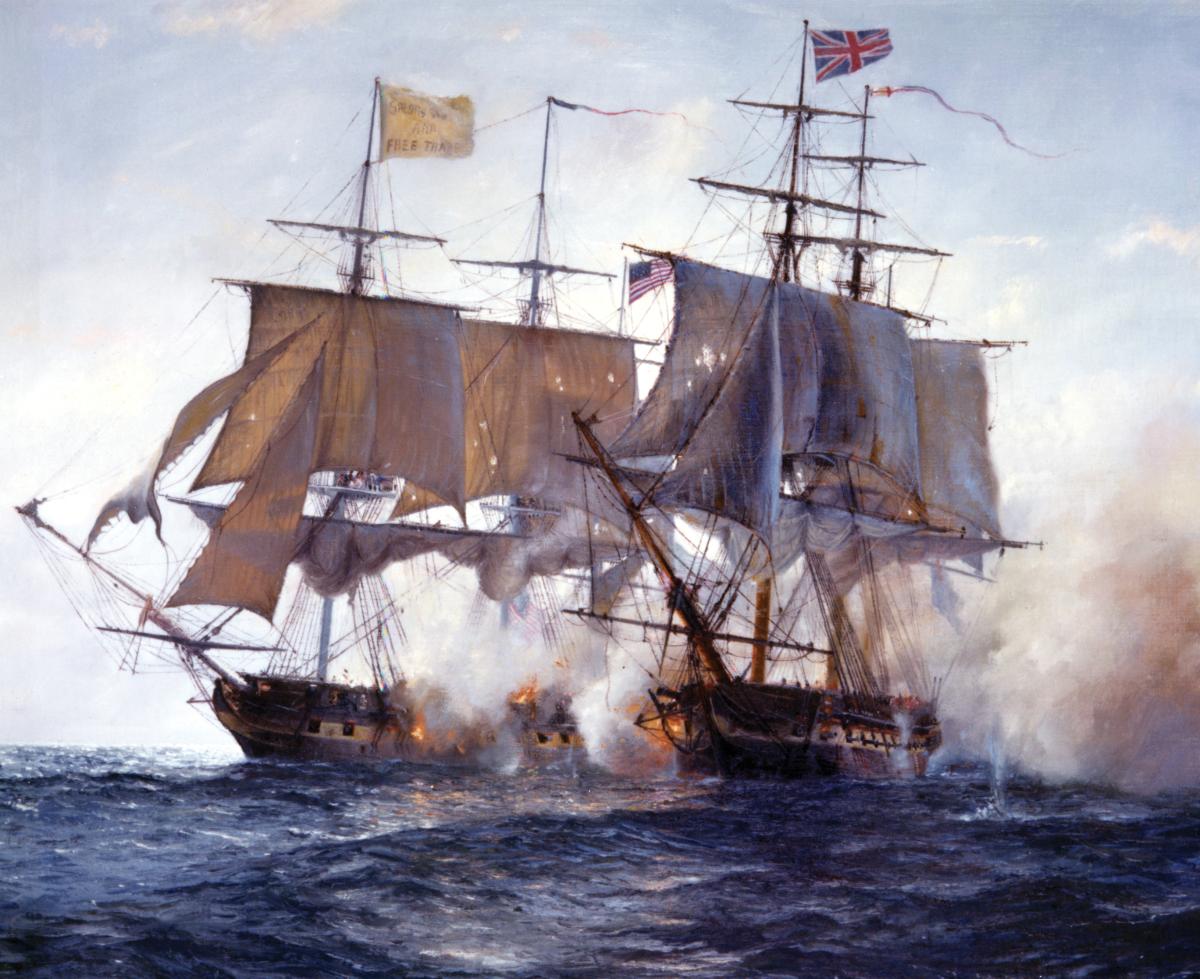This painting vividly depicts a dramatic naval combat scene between two 17th or 18th-century sailing ships, locked in close quarters and firing cannons upon one another. The water beneath them is a dark, turbulent blue, indicative of a rough and intense seascape. The sky is clouded, an almost white backdrop, contributing to an overall atmosphere of tension and conflict.

The ship on the right prominently displays a British flag, characterized by its blue field with red markings forming a cross and diagonal angles. Despite the intricate portrayal of the British flag, the ship itself appears to be weathered by the ongoing battle, with potential signs of fire damage. Conversely, the vessel on the left flies an American flag on its third mast, suggesting a historical context possibly rooted in the War of 1812, even though this detail might lend an imaginative twist given the anachronistic aspects.

Both ships are full-rigged, featuring the detailed rigging and hull designs emblematic of the era, akin to those of the famed USS Constitution. Overall, the scene captures the chaotic and perilous nature of naval warfare, with choppy waves and foggy, cloud-laden skies adding to the painting's dramatic intensity.